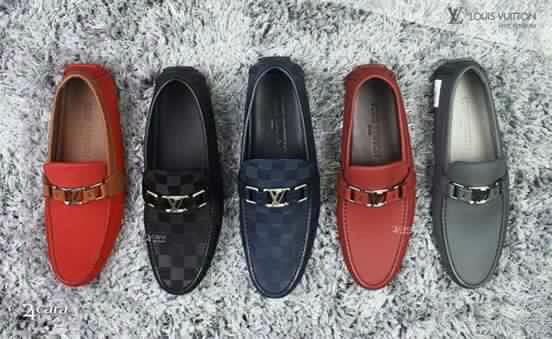The image displays an array of five single loafers, each belonging to the left foot, neatly arranged on a lush, shaggy gray carpet. All the shoes are crafted from high-quality leather and designed in a similar loafer style, exuding elegance and sophistication. The shoes feature different colors and distinctive hardware designs:

1. A deep burgundy-red loafer with a rich brown insole, adorned with a gold buckle at the top.
2. A black checkered-patterned loafer, displaying a darker and lighter shade of black, with a silver buckle and a black insole.
3. A dark navy blue checkered-patterned loafer, featuring alternating shades of blue, complemented by a silver Louis Vuitton buckle and a black insole.
4. Another red loafer, similar to the first in color, but this one has a gray insole and is elegantly finished with a gold buckle.
5. Finally, a gray loafer with a light gray insole, marked by a sleek silver buckle.

All shoes are presented on a plush gray shag rug, highlighting the luxurious material and craftsmanship of each loafer, emphasizing details like the fine stitching and hardware.